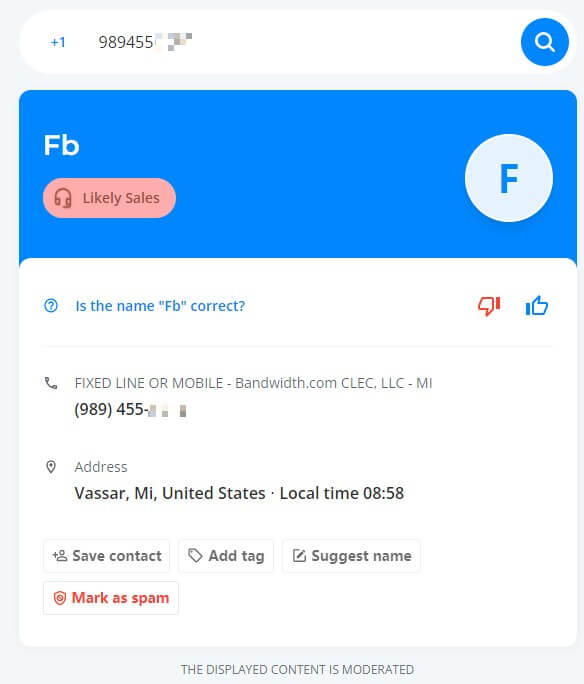The image captures a small screen interface, starting with a white search bar at the top. To the left within the search bar, it reads "+1" followed by the numbers "989455." On the far right of the search bar is a blue circle housing a white magnifying glass icon. Just above this search bar, a blue banner stretches across the top featuring the letters "F" and "B" in the top left corner.

Beneath the blue banner is a prominent red oval marked with "Likely Sales" alongside an icon of a headset. Below this, a white circle containing a blue "F" is visible. The majority of the remaining screen is white, showcasing blue text that asks, "Is the name FB correct?" Directly to the right of this query are two icons: a red thumbs-down and a blue thumbs-up.

Following this, the screen displays an image of a phone accompanied by the text "Fixed line or mobile" and additional identifiers: "bandwidth.com," "CLECLLCMI," and a phone number. Below this information, the address "Vassar, Michigan, United States" is listed, along with the local time, indicated as "8:58."

At the bottom section of the screen, options such as "Safe Contact," "Add Tag," and "Suggest Name" are available. Finally, at the very bottom, the name "Marcus Bam" appears in red text.